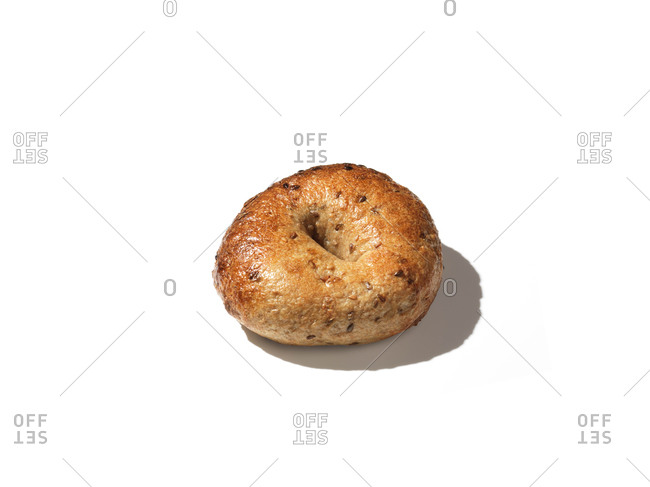This is a detailed photograph of a small, fully cooked bagel captured against a completely white background, enhanced with bright studio lighting. The bagel showcases the typical round doughy shape with a central hole, albeit not very pronounced, giving almost a solid appearance. The exterior boasts a glossy, golden-brown crust with a slightly crispy and shiny look, reflecting the bright lighting. This lighting also casts a distinct dark gray shadow extending to the lower right of the bagel, adding dimension to the image. Covering the bagel are black cooked sesame seeds, contributing to its multi-grain appearance. Overlaid on the photograph is a watermark of straight crisscross lines with either the logo "offset" or the number zero at each intersection. The "offset" logo features the word "off" with "set" flipped upside down and slightly translucent gray text.